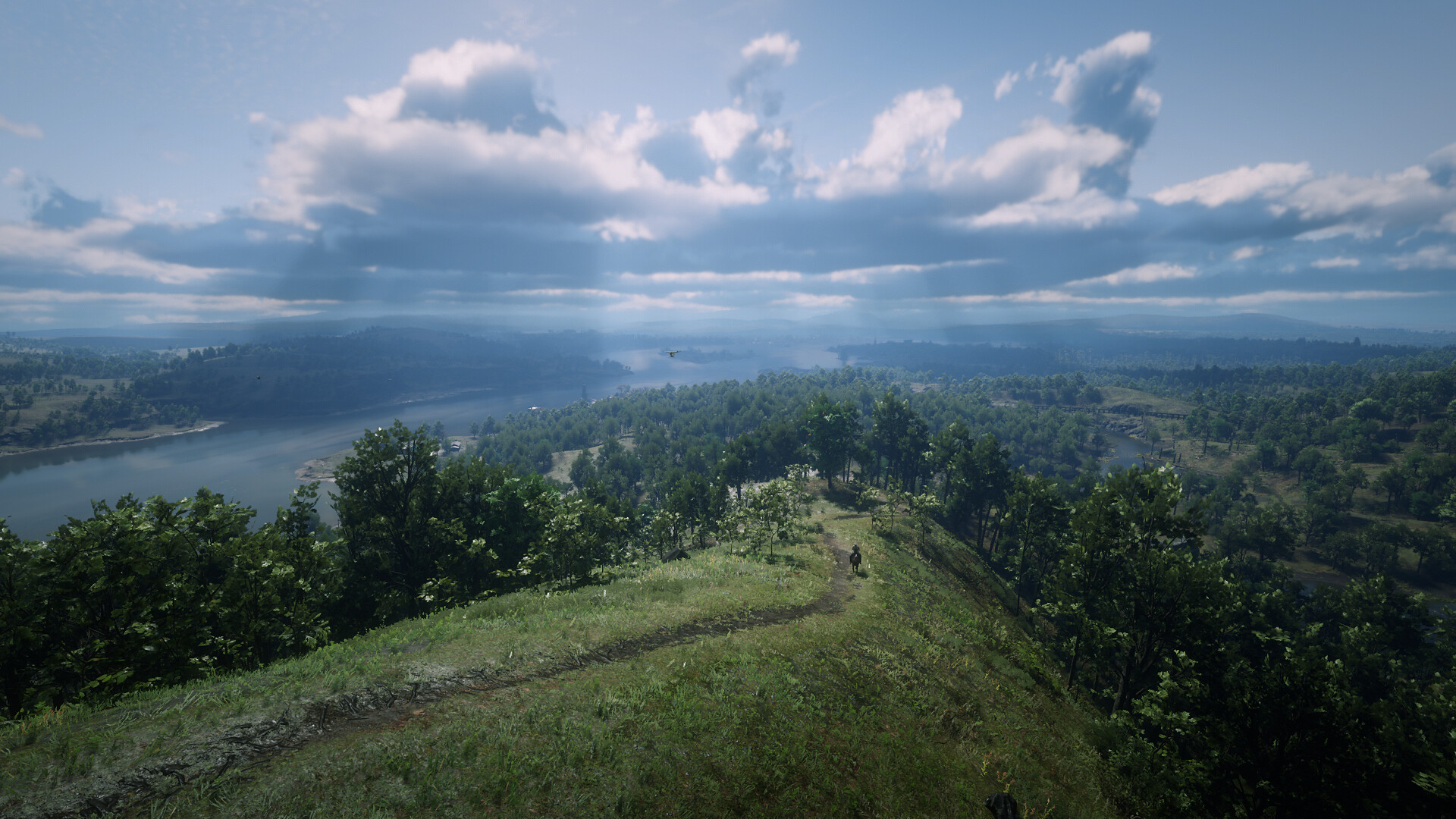A breathtaking aerial shot captures a winding path that ascends a steep hill, beginning in the lower left corner and meandering toward the center of the image. The hill's lush, green incline dominates the scene, offering a sense of serenity and solitude. On the left side of the path, a solitary tree stands tall, its presence adding depth and contrast to the landscape. Beyond the tree, a sizable, tranquil lake stretches into the distance, its serene waters reflecting the subtle hues of the sky. The sky itself is a vivid blue, adorned with the soft, idyllic edges of fluffy white clouds that spread across much of the horizon. The composition of the photo beautifully balances the natural elements, drawing the viewer's eye from the earthy path and verdant hill to the peaceful expanse of water and the vast, cloud-dappled sky.